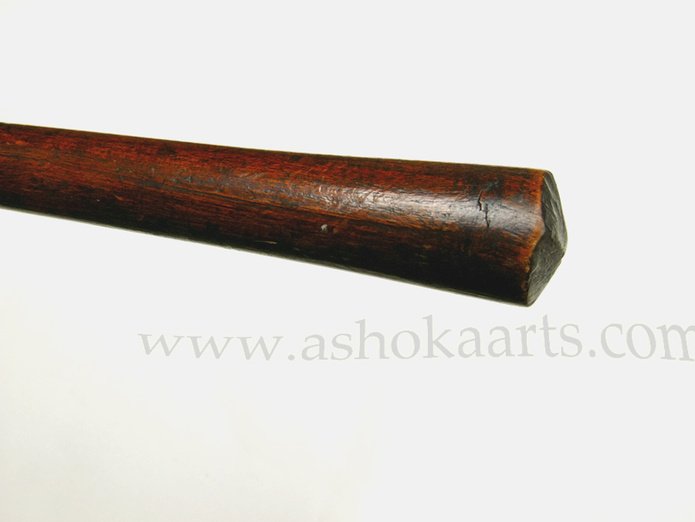The image is a full-color, rectangular photograph with a prominent horizontal orientation. Dominating the composition, a thick, round, wooden stick stretches from the left side, midway down the frame, extending nearly to the center and beyond. This piece of wood, which appears aged and worn with an amber hue, features a textured, rough end that is unevenly cut, suggesting it might be hand-crafted. The wood has a few dents and signs of wear, indicating its age and use. The background is a plain, light gray or white setting, highlighting the wood's details and texture. Beneath the image, the text "www.ashokarts.com" is watermarked, likely indicating the source or gallery associated with the photograph.